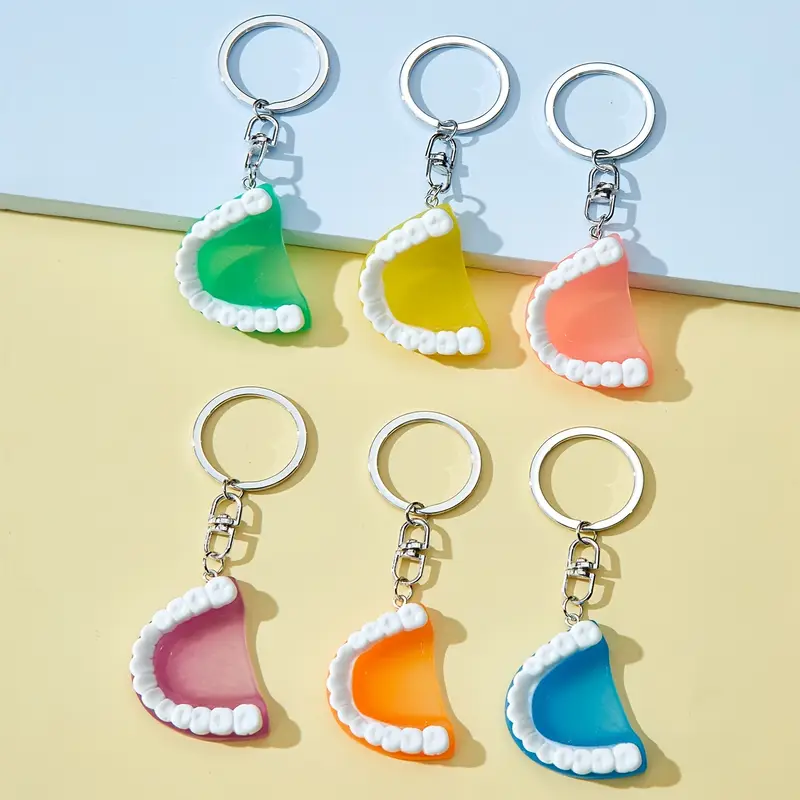This indoor color photograph showcases a collection of six keychains designed to resemble the upper jaw of human teeth, each unnaturally white and mounted on translucent plastic bases. Arranged in two neat rows of three keychains each, the top row features keychains with green, yellow, and pink plastic bases from left to right, while the bottom row consists of keychains with purple, orange, and blue bases in the same order. Each keychain is equipped with a silver hoop and a short silver chain connecting the teeth to the hoop. The background of the image is a two-toned surface with a light blue upper section and a sandy tan lower section, and shadows cast by the keychains are visible behind them.